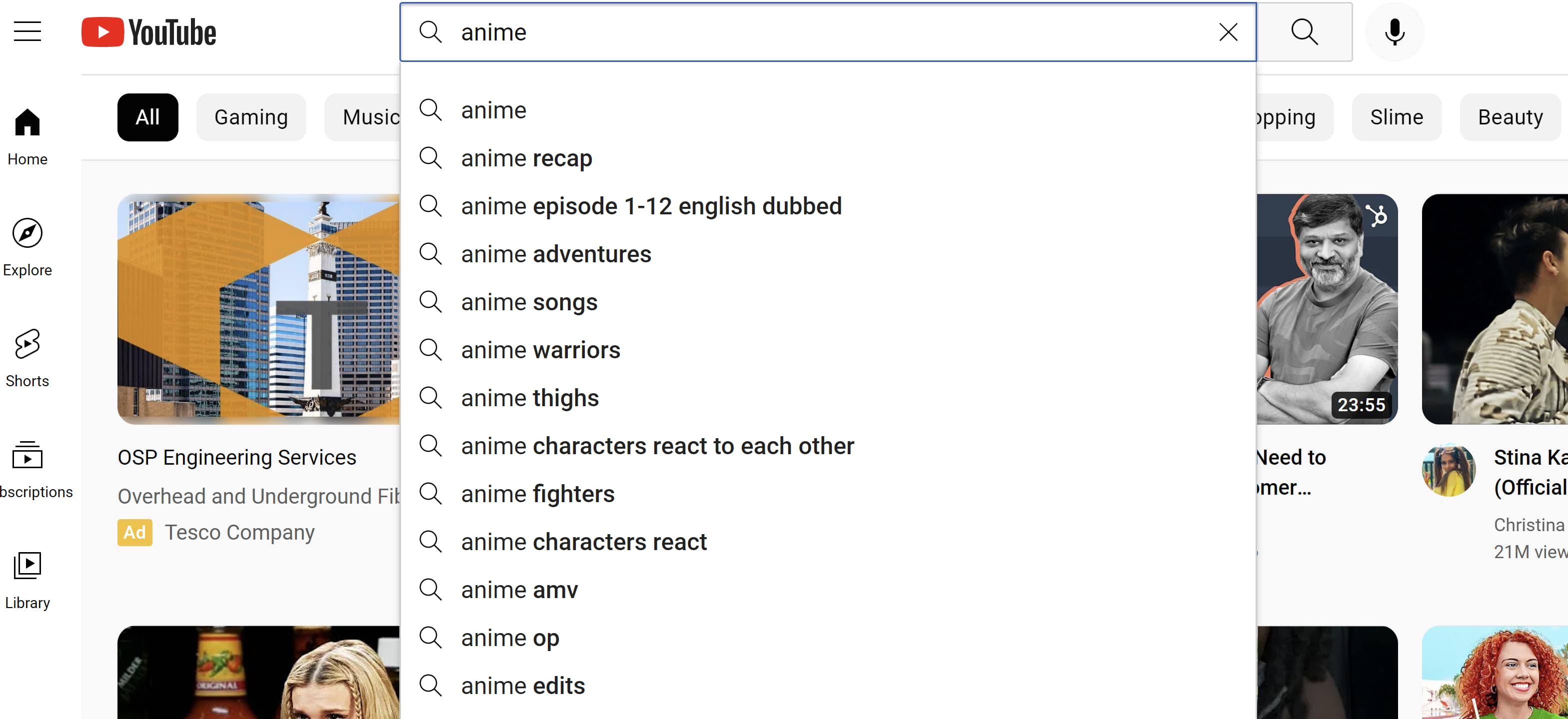The screen capture from YouTube displays the top toolbar prominently featuring the iconic red square with the play button, alongside the YouTube logo on the left. Positioned to the right of the logo is the search box with the word "anime" typed into it, indicating the user's search query. Adjacent to the search box are the magnifying glass icon and the microphone icon.

Beneath the search bar, a drop-down list reveals various autocomplete suggestions related to the search term "anime," including: "anime," "anime recap," "anime episode 1 through 12 English dubbed," "anime adventures," "anime songs," "anime warriors," "anime thighs," "anime characters react to each other," "anime fighters," "anime characters react," "anime AMV," "anime OP," and "anime edits."

On the left side of the screen, a vertical sidebar menu displays several icons: "Home," "Explore," "Shorts," and "Library." Below these main options, additional sections include "Descriptions" and "Library." Further categorization presents sections such as "All," "Gaming," "Music," "Shopping," "Slime," and "Beauty," providing a comprehensive view of the available navigation and content options on YouTube.